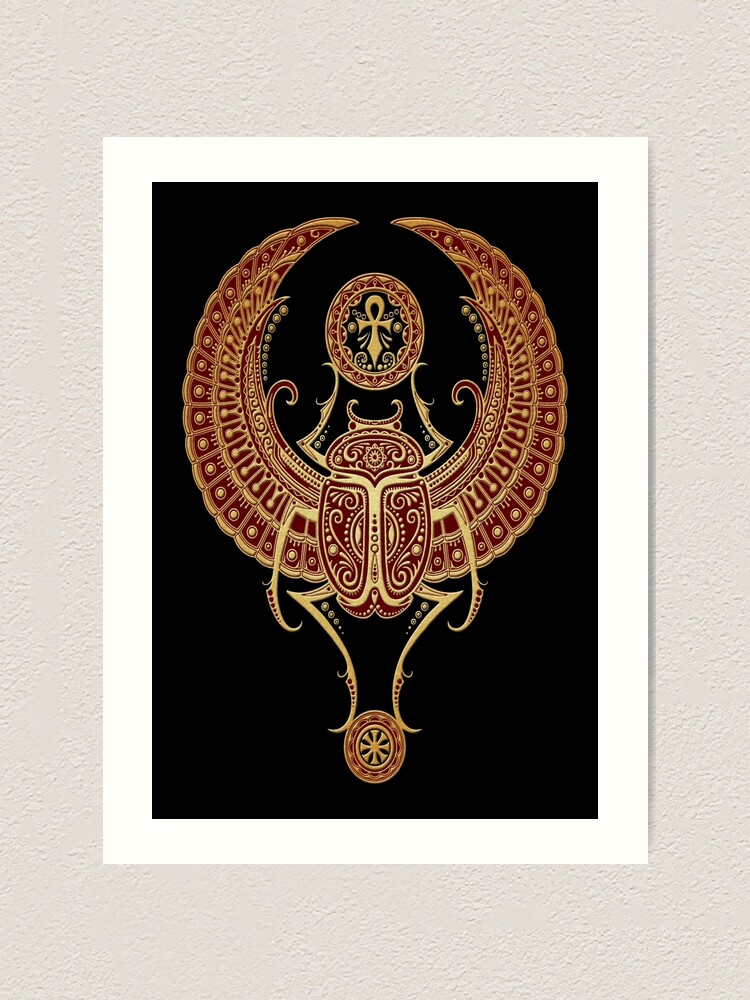The image depicts an intricate and luxurious piece of artwork, prominently featuring a stylized, ornate depiction of a beetle. The beetle has striking wings that arch upwards, almost meeting at the tips, with delicate gold and red accents creating a sense of opulence. Surrounding the beetle is a meticulously detailed design, replete with fine patterns of squares and circles, giving the artwork a unique and sophisticated appearance. The central image of the beetle is framed by a series of borders: a tan border closest to the artwork, followed by a white border, and then a black border, all set against a black surface background. The photograph appears to be taken from a direct overhead angle, emphasizing the intricate details and the careful composition of colors, including black, maroon, gold, white, and beige. This artwork, possibly a print or a poster, exudes a luxurious and majestic aesthetic, akin to an insignia or emblem, with a focus on the central beetle motif highlighted by the contrast of the rich background.